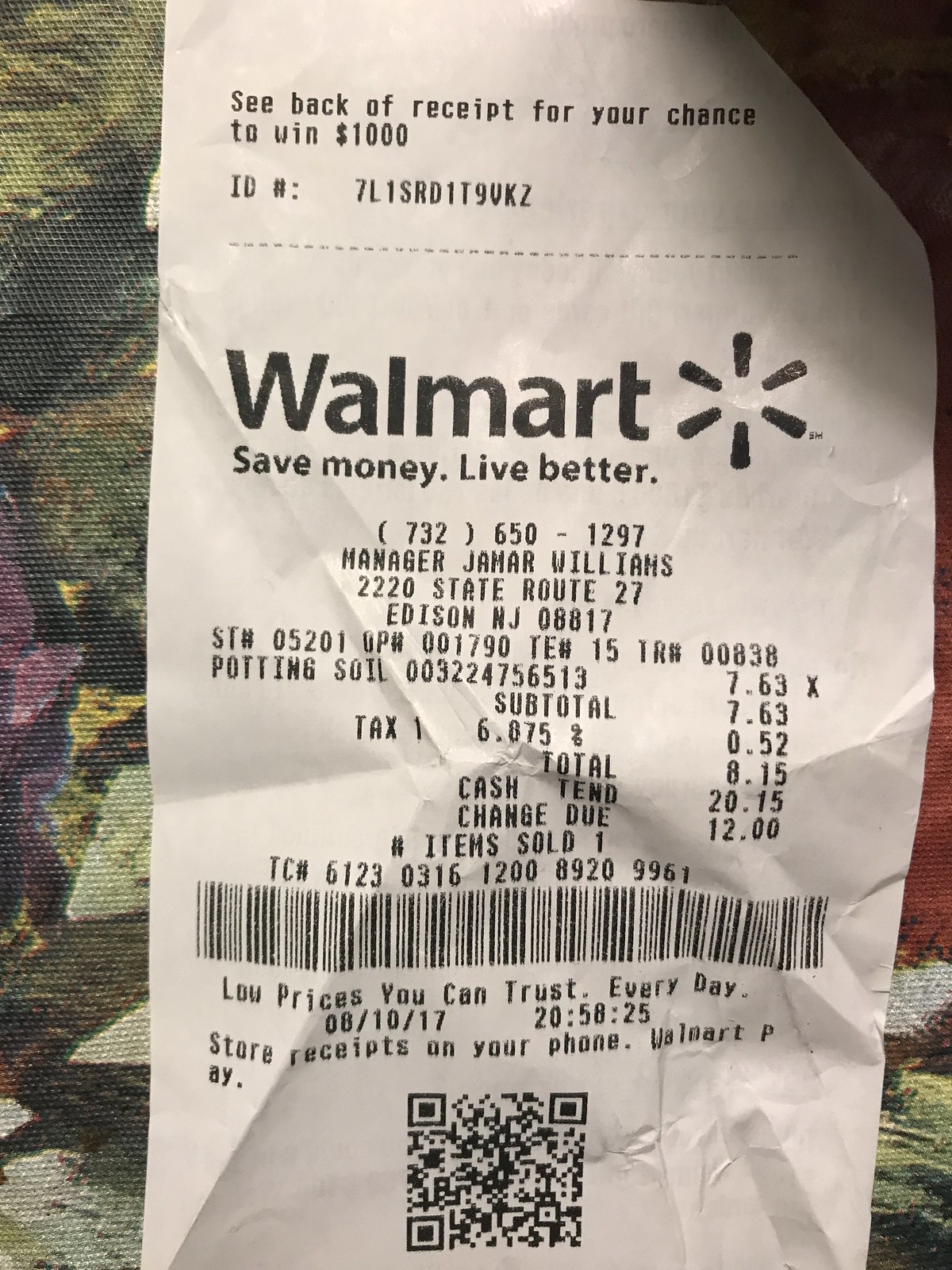This photograph showcases a detailed Walmart receipt placed against a vibrant, multicolored background featuring shades of white, blue, purple, and yellow. The receipt’s top left corner is slightly folded over. At the top, it mentions a promotional message: "See back of receipt for your chance to win $1,000" with an ID number "7L1SRD1T9QK2."

Beneath this, the Walmart logo is prominently displayed, with the tagline "Save money. Live better." All text on the receipt is printed in black. Detailed store information follows: 

- Phone number: (732) 650-1297
- Manager: Jamar Williams
- Address: 2220 State Route 27, Edison, NJ 08817
- Store identifiers: ST number 05201, OP number 001790, TE number 515, TR number 00838

The product listed is "Potting soil" with item code "003224756513," priced at $7.263. The receipt breaks down the financial details as follows:

- Subtotal: $7.263
- Tax (6.875%): $0.52
- Total: $8.15
- Amount tendered: $10.00
- Change due: $1.85

It notes that only one item was purchased, with a transaction code "TC number 61230316120089209961." A large barcode is positioned below this information.

The footer of the receipt includes the message "Low prices you can trust. Every day," along with the date and time of the transaction: "08/10/17 20:58:25." Additionally, it promotes digital storage of store receipts through "Walmart Pay."

A QR code is centered at the bottom of the receipt.